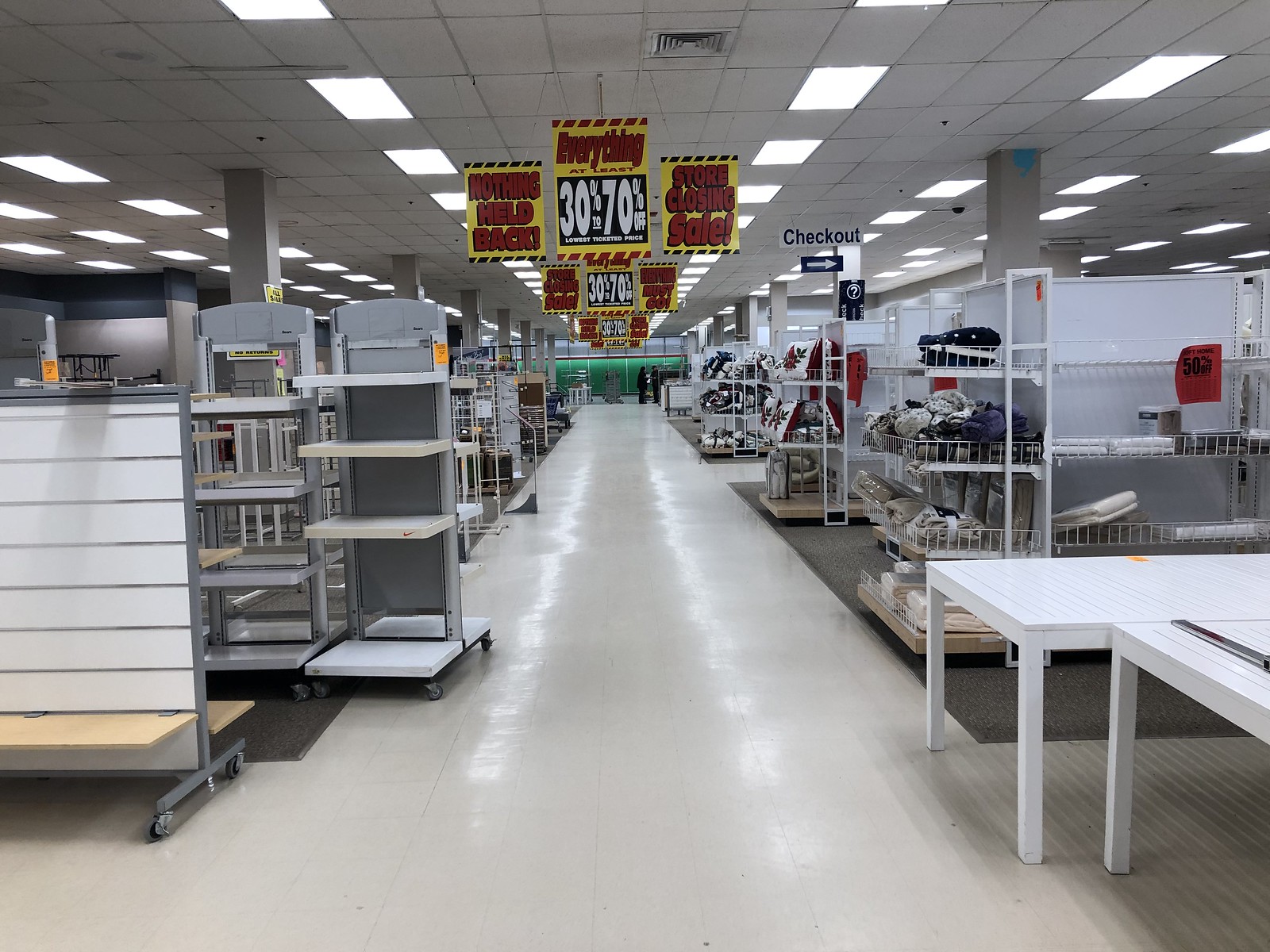The image depicts a store that is in the process of closing down, evident from the multitude of signs across the premises. Prominently, there are large, yellow signs with red writing that proclaim discounts ranging from 30% to 70%, and phrases like "Nothing Held Back" and "Store Closing, Everything Must Go." These signs are attached to the ceiling and scattered throughout the aisle. The floor is white linoleum, and the aisle shows a combination of white tables, rolling carts, and shelves on wheels, many of which are empty or sparsely populated with items such as towels, home décor, and pillows with tree designs. On the right side of the image, there is a white table and a rolling rack of clothing. Towards the back of the store, above an aisle, there is a sign in blue lettering that reads "Checkout" with an arrow pointing to the right. The lighting is from overhead fixtures, contributing to the stark, somewhat desolate atmosphere of a once bustling multi-market store now winding down its operations.